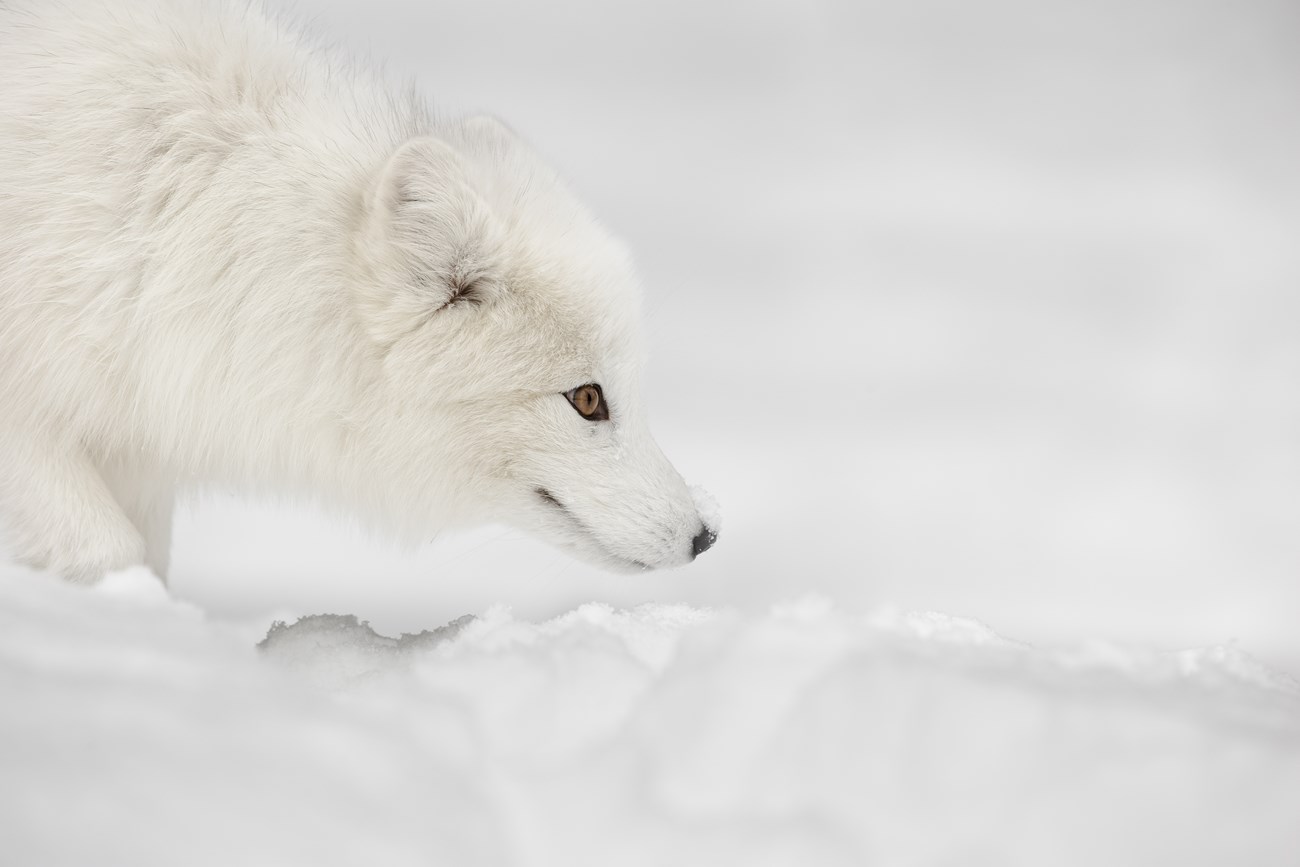The photograph is a horizontally oriented and highly detailed image capturing a serene winter landscape. The foreground and background are predominantly covered in textured, powdery white snow, with the background slightly blurred and tinged with shades of bluish white and lilac. 

Dominating the left side of the image is a beautiful white arctic fox, seen in profile, gazing intently to the right. The fox's right side is fully in focus, extending from the tip of its nose to just behind its front paws. The fox's dense, medium-long fur is a pristine white, with a few gray or black hairs interspersed, and a creamier tone than the surrounding snow, allowing it to stand out subtly against the backdrop.

Its ears are upright, rounded at the top, and contain minimal darker shading. The eyes are striking, with yellowish-amber irises and dark pupils, encircled by prominent black outlines. The fox’s small, black nose is dusted with snow, emphasizing its activity in the wintry setting. The fox’s expression is one of intense focus, its mouth firmly closed, as if it is intently tracking or contemplating something beyond the frame. The overall scene is peaceful and immersed in the serene stillness of a snowy environment, devoid of people or additional elements.